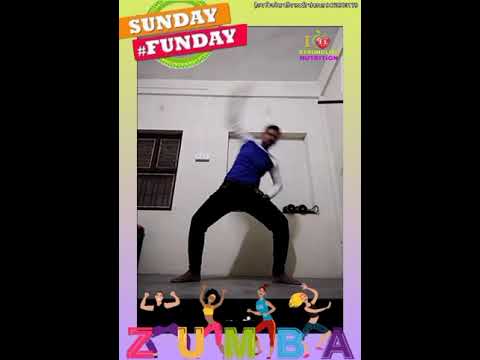This detailed image showcases a young Indian man engaged in what appears to be a lively dance routine, likely Zumba, as indicated by the colorful "Zumba" text at the bottom. He is on a gray cement floor with a white wall behind him, where a white shelf, seemingly holding weights, is mounted. The man is dressed in an eye-catching outfit: a tight, long-sleeved shirt with a blue body and white sleeves, paired with black jeans or sweatpants and bare feet. His pose is dynamic; he's crouched down slightly, with legs spread apart, one knee bent more than the other. His right arm rests on his thigh while his left arm is raised, seemingly in motion, as suggested by a slight blur.

The upper left side of the image features the phrase "Sunday fun day" in a stylized text, with "fun day" accompanied by a hashtag, enclosed in an orange and red box with a green ring. A black-bordered window is present on the left side of the image, contributing to the setting's somewhat rundown feel. Additionally, whimsical cartoon figures of dancing women are displayed beneath the Zumba text, reinforcing the theme of energetic exercise. The overall image is bordered with yellow on the top and purple on the bottom, adding a vibrant frame to this lively scene.